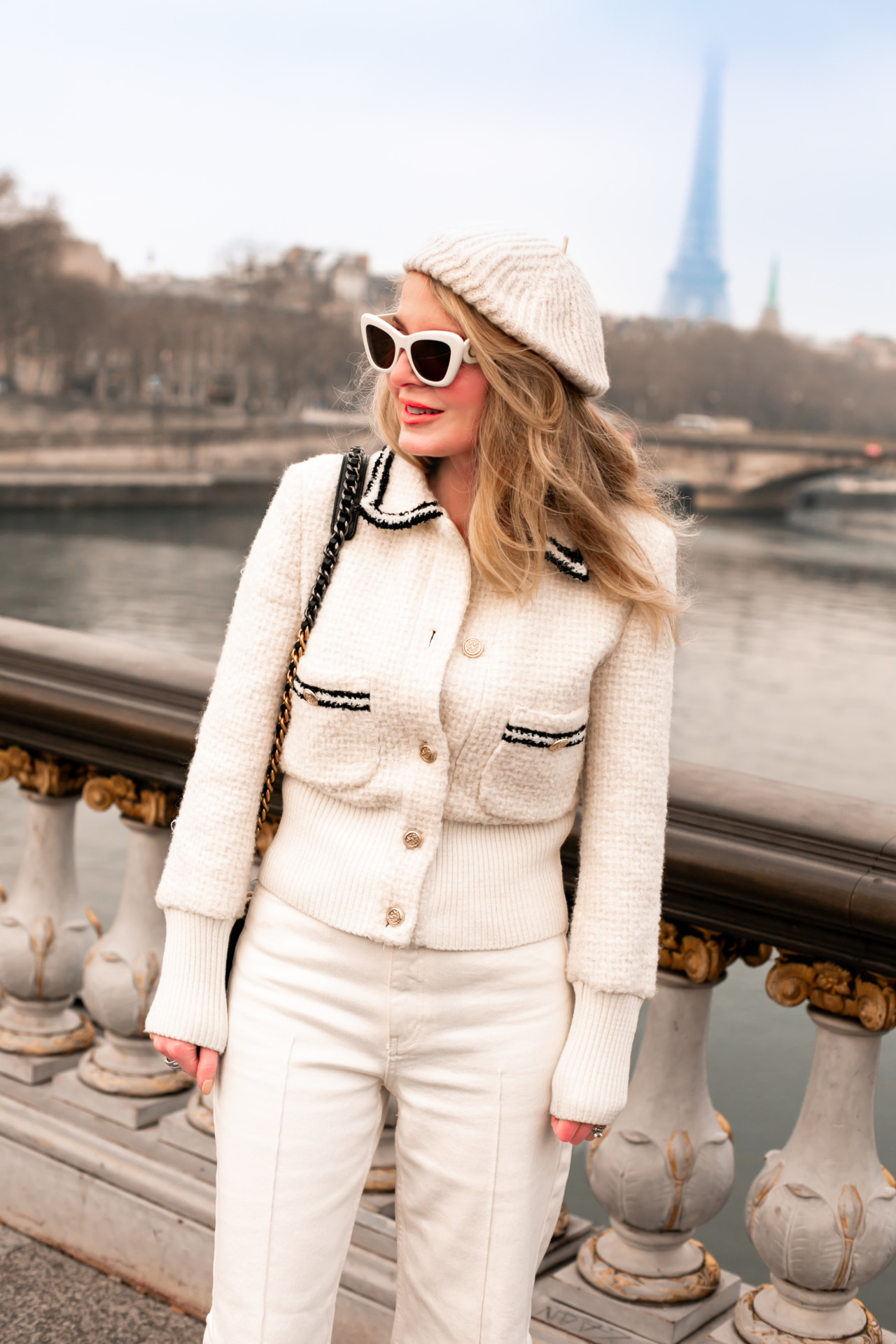The image showcases a blonde woman outdoors, smiling and looking slightly to the left. She is dressed in a fashionable, all-white outfit consisting of a white beret, white-framed sunglasses with dark lenses, a white sweater with black trim on the collar and pockets, and white pants. Her blonde hair flows down past her neck, and she carries a handbag on her right shoulder. The setting includes a stone balustrade overlooking a body of gray water, with the iconic Eiffel Tower visible, though out of focus, in the hazy, light blue sky background. In the top right corner of the image, blurred buildings can be seen. The overall scene evokes a sense of travel or fashion, with the woman appearing to be a tourist enjoying a moment in Paris.